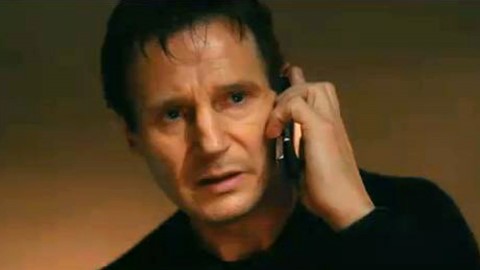The image appears to be a still from the movie "Taken," featuring the actor Liam Neeson. Set in a rectangular frame with a horizontal orientation, the background is predominantly dark brown, lightening slightly towards the bottom. Neeson, a white man in his mid-fifties with short brown hair and dark eyes, is shown from his shoulders upwards. His hair slightly tousled and his high forehead visible, he exudes a worried and concerned expression. Neeson's head is inclined from right to left, his mouth partially open as if mid-sentence. He wears a long-sleeve black shirt with a crew or round neck. His left hand is raised, holding a small cell phone with a black edge and possibly a tan or light brown body, to his left ear. The image emphasizes his intense, concerned demeanor as he converses on the phone. There is no text present in the image.